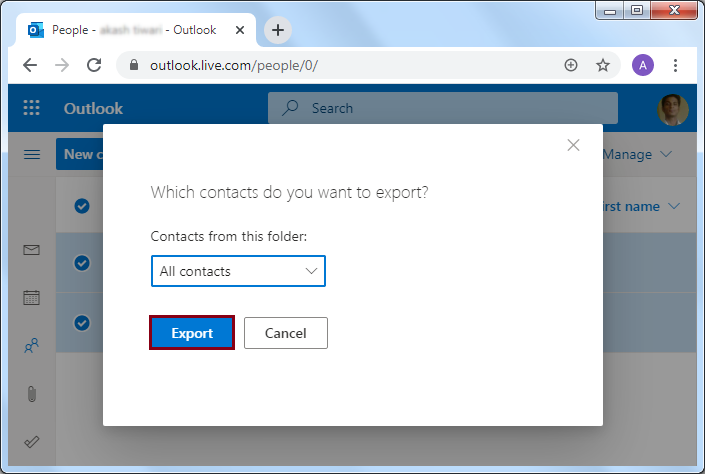The image showcases an Outlook email interface focused on the "People" tab. A white dialog box has popped up, indicating an operation to export contacts. The dialog box presents the prompt "Which contacts do you want to export?" followed by smaller text reading "Contacts from this folder:", and a dropdown box encased in a blue outline labeled "All contacts," which can be adjusted to filter the contacts. Below this dropdown are two buttons: "Export" in blue and "Cancel" in white.

In the upper part of the image, next to the "People" tab, there is an 'X' icon to close the tab, a '+' icon to add a new tab, and buttons to navigate back, refresh the page, and more. The URL is outlook.live.com, showing the user's profile icon as an "A" in purple on the far right. Beneath the URL bar, there is a search field for Outlook.

Though partially obstructed by the white dialog box, there appears to be a blue bar with white text reading "New contact." Additionally, three checkmarks are visible in the main interface, but their associated text is unreadable due to the overlaying dialog box.